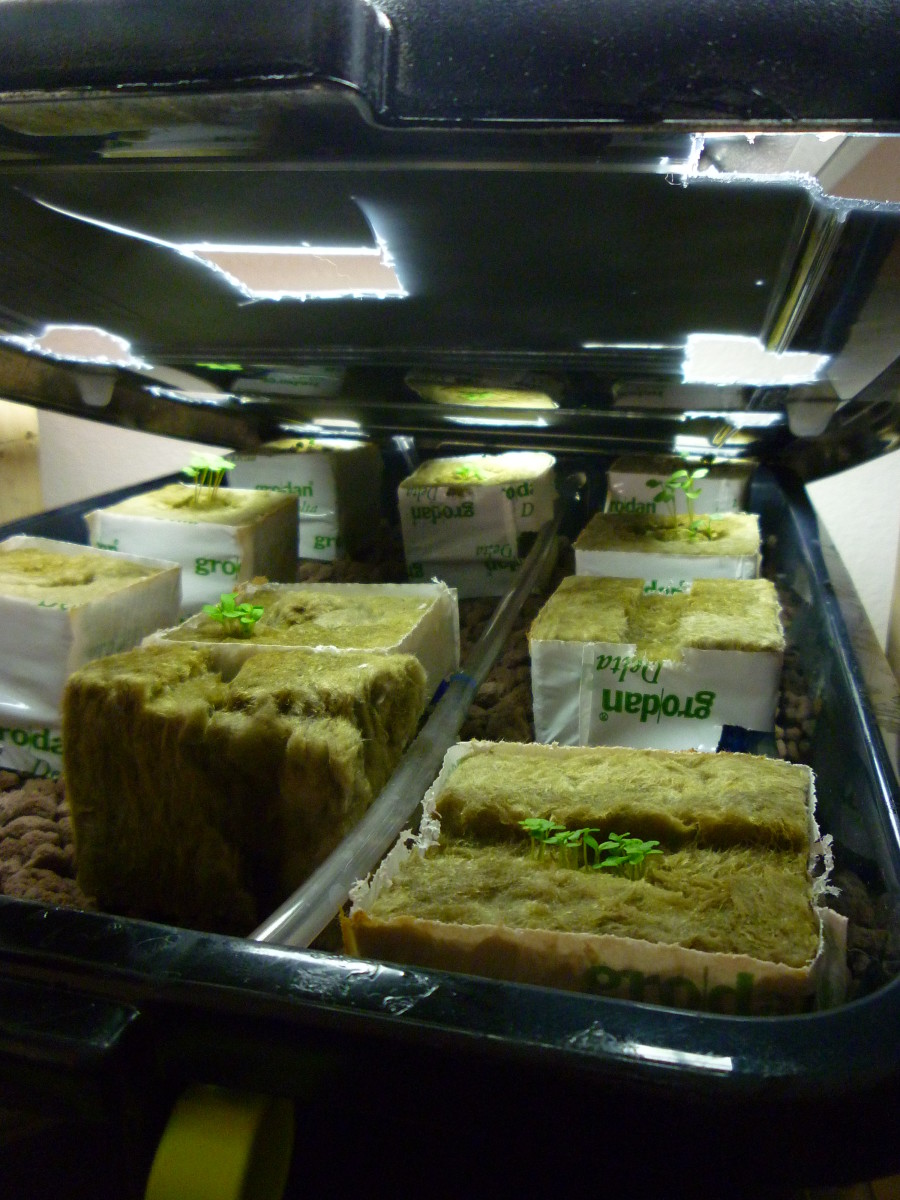The image depicts an indoor gardening setup, featuring a black plastic container with its lid opened to reveal a total of ten small plants. Each plant is sprouting from blocks that appear to be spongy and have a yellowish-brown color. These blocks are wrapped in white paper with green writing, which spells out "G-R-O-D-A-N," though the positioning of the writing varies, with some words appearing upside down. The blocks are arranged in rows: three on the left, two in the center, and four on the right-hand side. A plastic tube runs between the plants, likely for irrigation. Light is shining down from the top of the container, supporting the growth of the green seedlings that emerge from a fibrous material used as the growing medium. The walls behind the setup are white, providing a clean, controlled environment for the plants.